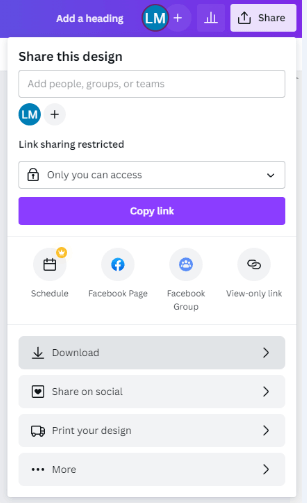Screenshot of a Canva Design Sharing Options Interface:

The image is a screenshot displaying Canva's design sharing and upload options on a user's phone. At the top, there's a blue header bar with white text that reads "Add a heading." To the right of this heading are the user's profile picture marked with the initials "L.M.," a white plus symbol, and a white graph icon.

Below the header, the interface features a section in black text on a white background. It includes an upload icon and the word "Share." Beneath this, the text "Share this design" prompts the user to type in names within a white bar designed for this purpose. This section is followed by the user's profile picture again along with a plus icon, indicating the option to add more people.

The next section contains black text that states "Link sharing restricted," with a corresponding white bar that reads "Only you can access" accompanied by a lock icon and a dropdown menu. Below this, there is a prominently displayed purple or blue button containing the white text "Copy link," followed by a small gray bar.

Subsequent options are presented for scheduling posts (marked by a crown icon), sharing on a Facebook Page (with the Facebook icon), Facebook Group (with the Facebook Groups icon), and creating a view-only link (illustrated with two interlinked chain icons).

At the very bottom of the interface are four wide gray option bars with black text and right-facing arrows on their right sides. From top to bottom, these options read: "Download" (with a download icon), "Share on social" (with a heart inside a square), "Print your design" (with a truck icon), and "More" (represented by three black dots).

This annotated interface provides a comprehensive overview of sharing and distribution settings within Canva's design platform.